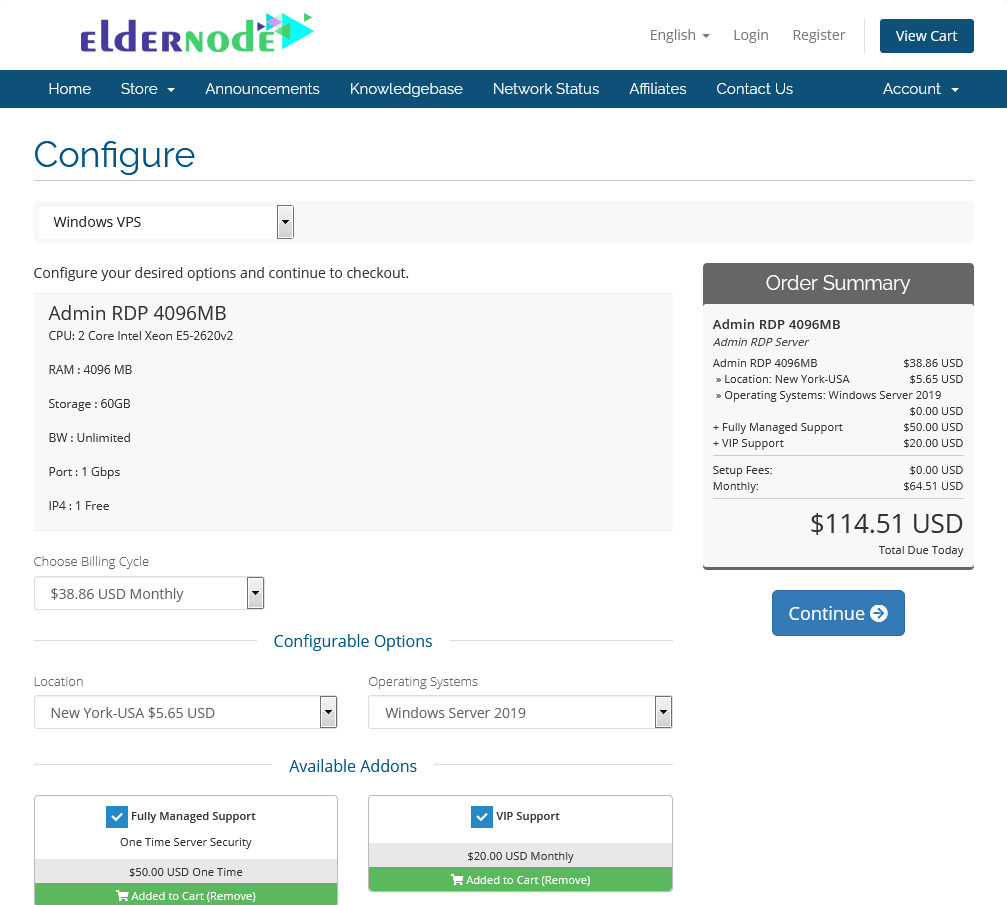In the image, there is a prominently featured section at the top labeled "ElderNode" in distinctive purple and green colors. To the right side, the words "English login register" are presented in gray text. Adjacent to this, a blue box with white text displays the label "ViewCard". Additionally, a blue horizontal banner spans the top of the image.

Beneath this banner, a navigation bar provides links in white text labeled "Home, Store, Announcements, Knowledge Base, Network Status, Affiliates, Contact Us," and "Account". Further down, a large blue heading reads "Configure", indicating the start of the configuration section.

In the subsequent section, titled "Windows VPS", users are prompted to "Configure your desired options and continue with checkout." Below this prompt, details of the service are provided, including:
- Admin RDP with 4096 megabytes of RAM
- A CPU featuring a two-core Intel Xeon processor
- 4096 megabytes of RAM
- 60 gigabytes of storage
- Unlimited bandwidth (BW)
- A one-gigabit port
- An IP address listed as 413

To the right, an order summary reiterates the Admin RDP with 4096 megabytes of RAM, along with a detailed pricing breakdown leading to a total of $114.51 USD, which is due today. At the bottom of this section, a blue box with white text prompts the user to "Continue".